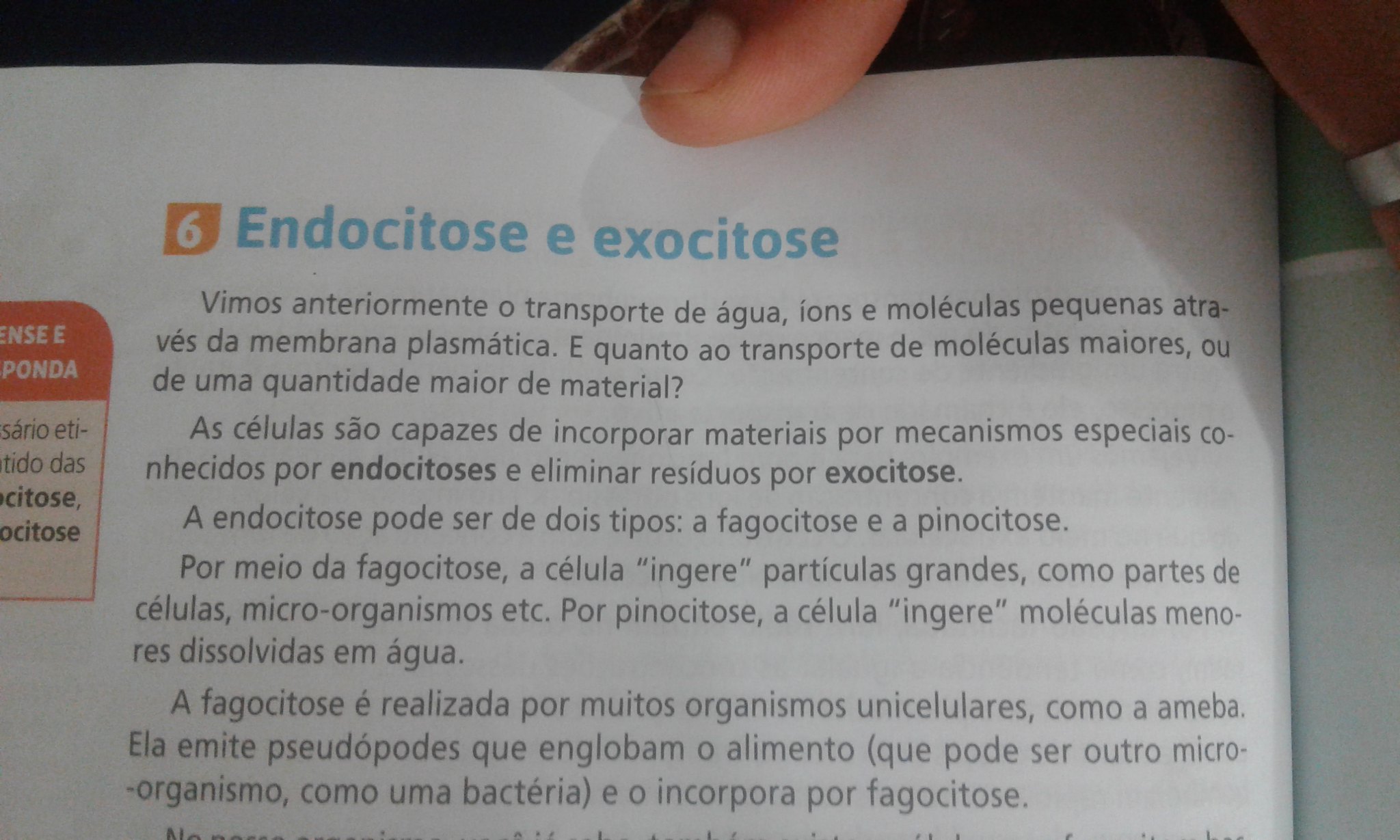The rectangular photograph captures a close-up of a person's hand holding open a page of a book or magazine. The image focuses on the tips of a few fingers, with one finger adorned with a silver band. The page features predominantly black text on a white background. In the upper section, an orange square block contains some black and white print, which appears to be in a foreign language, potentially Spanish or Portuguese. Above this, another orange block bears a white number six. The main heading in blue reads "Endocytosis Exocytosis," while another legible portion of the text includes the phrase "de agua," meaning "of water." The intricate details of the text remain unreadable, but together these elements create a visually compelling snapshot of a moment mid-read.